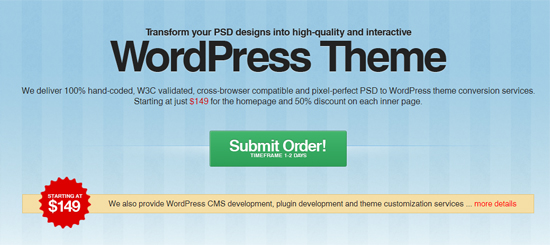**Image Description: WordPress Theme Promotion Ad**

The image is a promotional banner for a WordPress theme conversion service. It features a large blue rectangular box as the background. Centered within this box is the primary heading, "Transform Your PSD Designs into High-Quality and Interactive WordPress Themes", written in bold black text. Beneath this heading, "WordPress Theme" is prominently displayed in even larger, bold black font.

Below the titles, a detailed description informs potential customers about the service: "We deliver 100% hand-coded, W3C validated, cross-browser compatible, and pixel-perfect PSD to WordPress conversion services starting at just $149 for the homepage, with a 50% discount on each inner page."

Towards the bottom of the image, a green "Submit Order!" button invites users to take action. Adjacent to this, a red circular badge with star-like tips highlights the starting price, "$149", drawing special attention to the offer. A yellow banner runs across the bottom of the image, containing additional services offered, written in red: "We also provide WordPress CMS development, plugin development, and theme customization services. More details."